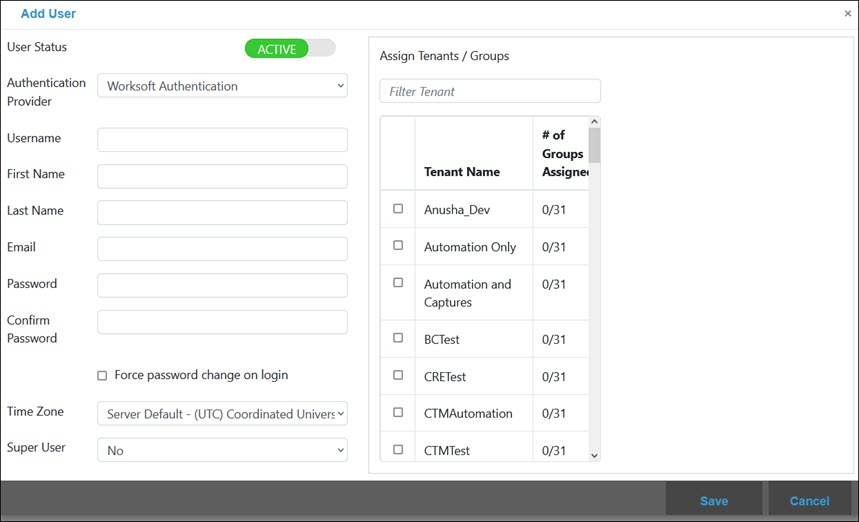The image showcases a highly minimalist user interface designed for adding a user to a system. The interface sits against a pristine white background, and at the very top, the heading "Add User" is prominently displayed. Below this heading, the form is divided into various sections that need to be filled out. These sections include fields for user status, the authentication provider, username, first name, last name, email, password, and password confirmation. 

Additionally, there is a checkbox available to mandate a password change upon the user's first login. Two dropdown menus are included: one for selecting the time zone and the other for designating a super user.

To the right of this form, there is a panel labeled "Assign Tenants/Groups." This section features a search bar that allows filtering by tenant. Below the search bar is a table with three columns. The first column contains checkboxes, all of which are currently unchecked. The second column is labeled "Tenant Name" and lists multiple tenant names. The third column is titled "Number of Groups Assigned," where each entry shows a fraction indicating '0 out of 31'.

At the very bottom of the interface, there are two actionable buttons to either save the newly added user or cancel the operation.